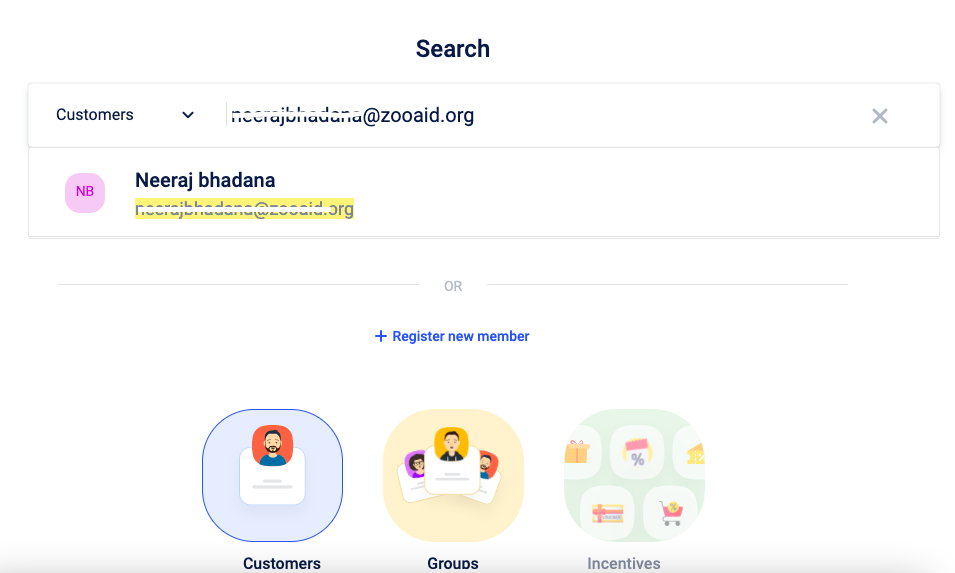Screenshot Description:

The screenshot displays a search interface, likely from a website accessed via a desktop or laptop, given the absence of typical mobile app icons at the top. Centered prominently at the top in large black text is the word "Search." Below this, on the left-hand side, is the word "Customers," accompanied by a downward arrow indicating a drop-down menu for additional selection options.

In the center of the screen, there is a partially redacted email address, which remains discernible as "neerajbhadana@zooegg.org." To the right of this email is an 'X' button, presumably to close or delete the entry. 

Beneath the email, a logo displaying the initials "NB" is present, followed by the name "Neeraj Bhadana," written in lowercase black text. The web address, "zooegg.org," is highlighted in yellow but has been struck through with a white line, suggesting an attempt at redaction.

A horizontal line marks a section break, below which there is a line of text reading "line - line" in light blue, adjacent to a blue plus sign. Further down, the interface lists three options for user roles or sections: "Customers," "Groups," and "Incentives." Notably, "Incentives" is greyed out, indicating it is not currently selectable.

To the left in the first option box, there is a circular logo featuring a person in the center.

This descriptive caption aims to encapsulate the visual elements and layout of the interface presented in the screenshot.